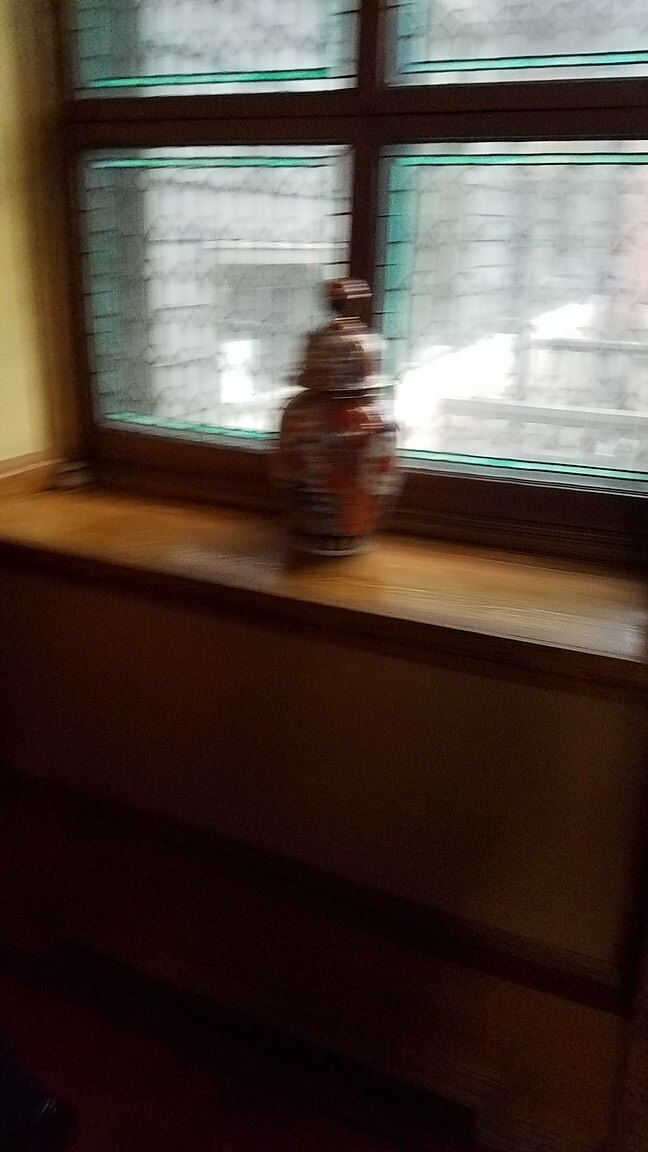A vertically-oriented, low-light photograph captures a slightly blurred scene focused on a window with four panes. Light streams through the window, illuminating a distinctive urn positioned on the windowsill. The urn, reminiscent of a fire hydrant in shape, features an ornate design. Its lid, a gold-colored sphere atop an upside-down bowl, contrasts with the vibrant red lower section of the urn, which is adorned with a shield emblem on the right side. The window frame is outlined with a turquoise border, adding a pop of color to the otherwise subdued light yellow wall visible in the upper left corner. The lower part of the image descends into dark shadow, shrouding the scene in a mysterious aura.